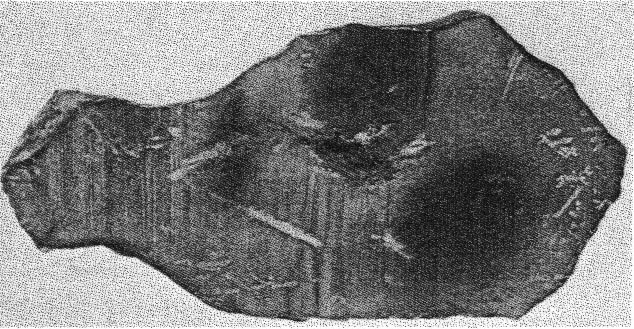A high-resolution X-ray image showcases an ancient piece of fabric recovered from an archaeological dig, undergoing analysis for age and origin. The background features a gray and white pixelated pattern, giving a scientific context to the study. The fabric in question appears to be a segment of a woman’s dress, with evident areas of wear over time. Light filters through the more delicate, frayed sections of the cloth, while denser regions remain opaque. Detailed designs resembling twigs or flowers are intricately woven into the fabric, hinting at its original aesthetic and cultural significance. The X-ray reveals not just a piece of cloth, but a rich tapestry of history and craftsmanship.